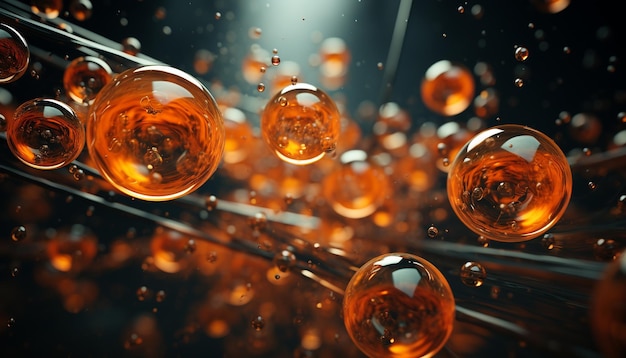This is a captivating action shot from an artist's unique perspective, taken from underneath what looks like a spilled glass, capturing droplets as they descend. The droplets, in varying sizes, range in color from light brown to amber, reminiscent of tea or soda. This up-close image makes you feel like you're lying beneath the scattering liquid, watching in slow motion as the droplets fall towards you, almost inciting an urge to close your eyes. Larger, clearer droplets are in the foreground while smaller ones and a variety of scattered marbles, reflecting light, populate the blurry background. Among these, thin, black skewer-like rods slice through the scene, all directed towards a central light source that beams from the top middle of the image. The background remains jet black, heightening the drama and contrast of the descending spears and marbles, giving the entire composition an otherworldly, almost atomic feel.